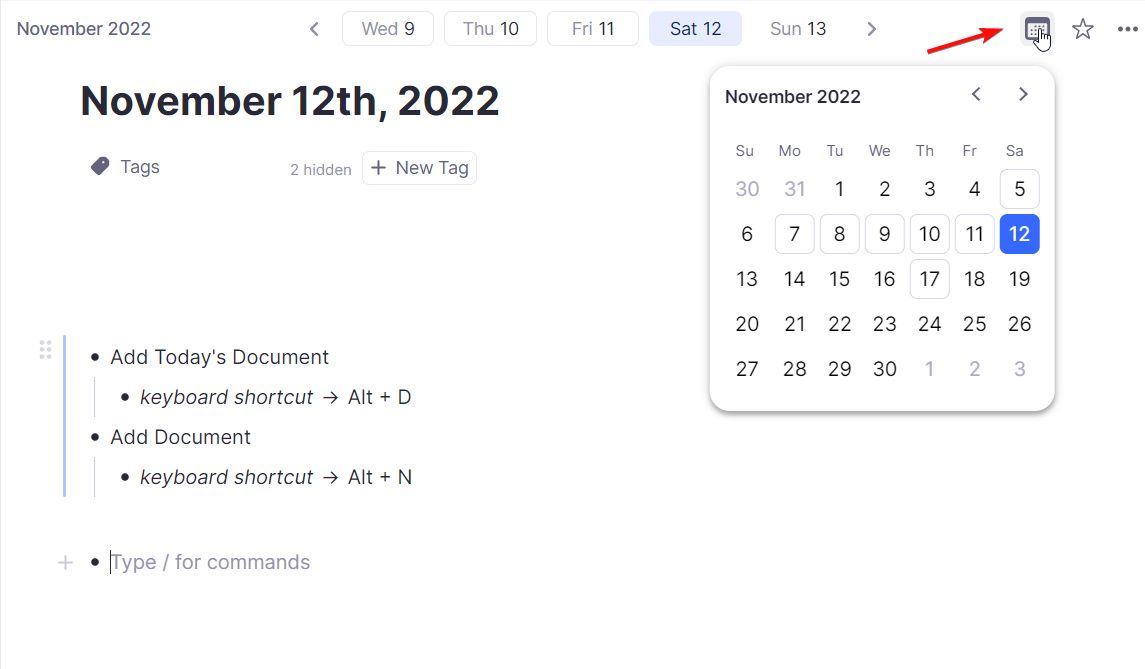This screenshot, displayed in portrait mode, captures a user interface presumably from a document or task management application, dated November 22nd, 2022.

The central feature of the image is a pop-up calendar with several elements annotated and highlighted:

1. **Current Date:**
   - The upper left corner of the screen prominently shows the date as "November 22nd, 2022".

2. **Day Buttons:**
   - At the top of the calendar, buttons for specific days are displayed. These include:
     - Wednesday, the 9th
     - Thursday, the 10th
     - Friday, the 11th
     - Saturday, the 12th (highlighted)
     - Sunday, the 13th
   
3. **Highlighted Dates:**
   - The date "Saturday, the 12th" is highlighted.
   - The calendar itself shows boxes around several dates: 5th, 7th, 8th, 9th, 10th, 11th, 12th, and 17th.

4. **Annotations:**
   - A red arrow points to a calendar, apparently initiating the display of this pop-up.

5. **Left Column Info:**
   - On the left side, "November 12th, 2022" is noted.
   - Below this, there are tags listed: "Two Hidden," "New Tag".

6. **Keyboard Shortcuts:**
   - The bottom section details keyboard shortcuts:
     - "Add today's document": Alt + D
     - "Add document": Alt + N

The screenshot seems to depict a potentially complex interface for scheduling or document tagging, with several dates marked, suggesting planned activities or document entries on those specific days.